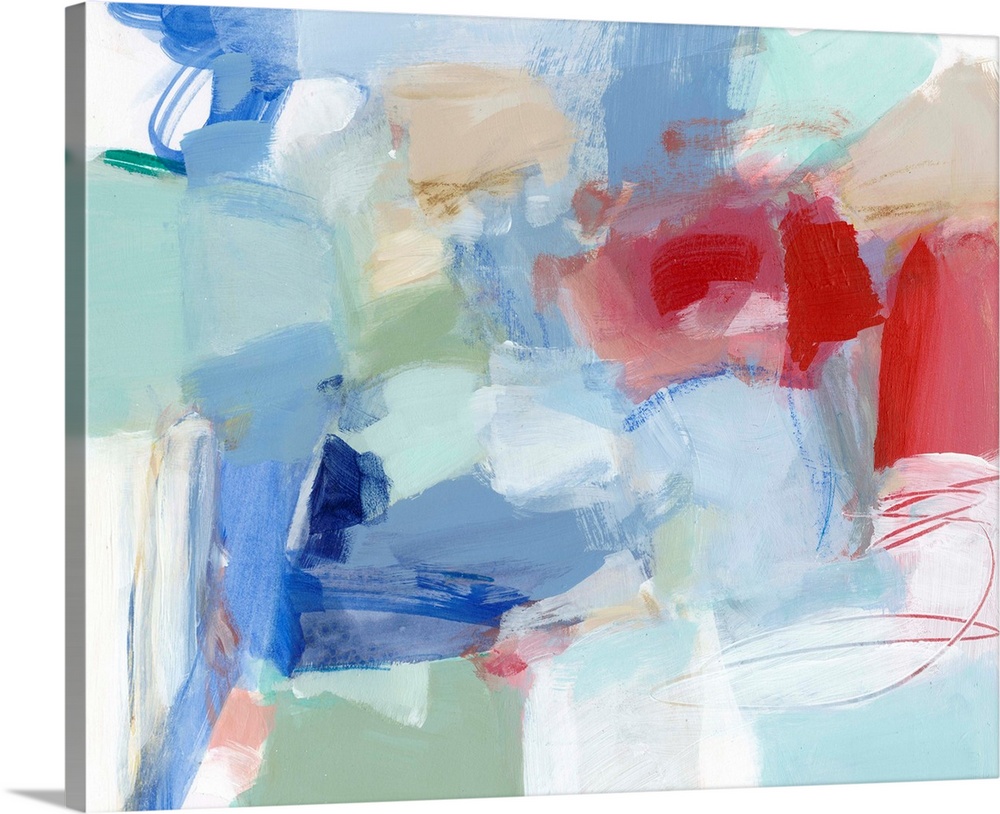This image features an abstract painting on a rectangular canvas, viewed from a slightly angled perspective that reveals the edges and the shadow behind the canvas. The composition is a vibrant, chaotic array of overlapping paint splotches and streaks, dominated by various shades of blue—approximately four distinct tones. Reds, including spirally red lines, mingle with greens, whites, browns, beiges, and cream colors across the surface. These colors create a complex, textured pattern with no discernible order, enhanced by thumbprint-like shapes embedded within the abstract layers. The overall effect is a dynamic, multi-layered visual experience that captures the spontaneous energy of the artist’s strokes.